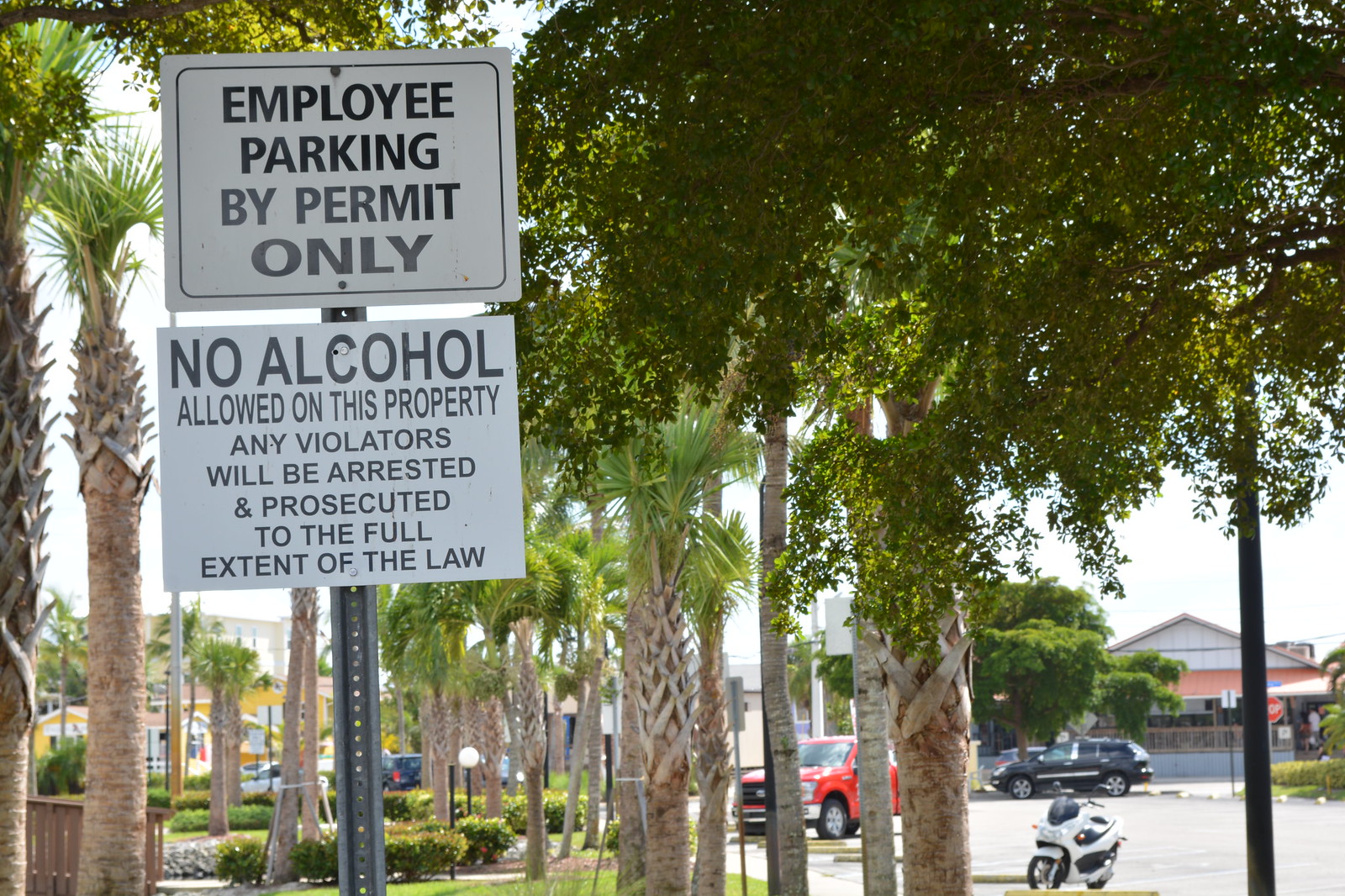In the foreground of the image, a metallic pole holds two rectangular white signs with black text. The top sign, bordered by a thin black line, reads "EMPLOYEE PARKING BY PERMIT ONLY," while the lower sign states "NO ALCOHOL ALLOWED ON THIS PROPERTY. ANY VIOLATORS WILL BE ARRESTED AND PROSECUTED TO THE FULL EXTENT OF THE LAW." Behind this signpost, a landscaped area showcases a manicured lawn with green grass interspersed with brown mulch patches. Various bush and palm trees populate the mulch, all leading down to a parking lot filled with an assortment of vehicles, including a red truck, a black SUV, and a white motorcycle. The backdrop of the scene includes some buildings and hints of other trees. There's also a ramp visible on the bottom left side of the image, its railing the only part clearly seen. The presence of palm trees suggests that this image might have been taken in a location with a warm climate, such as Florida or Los Angeles.